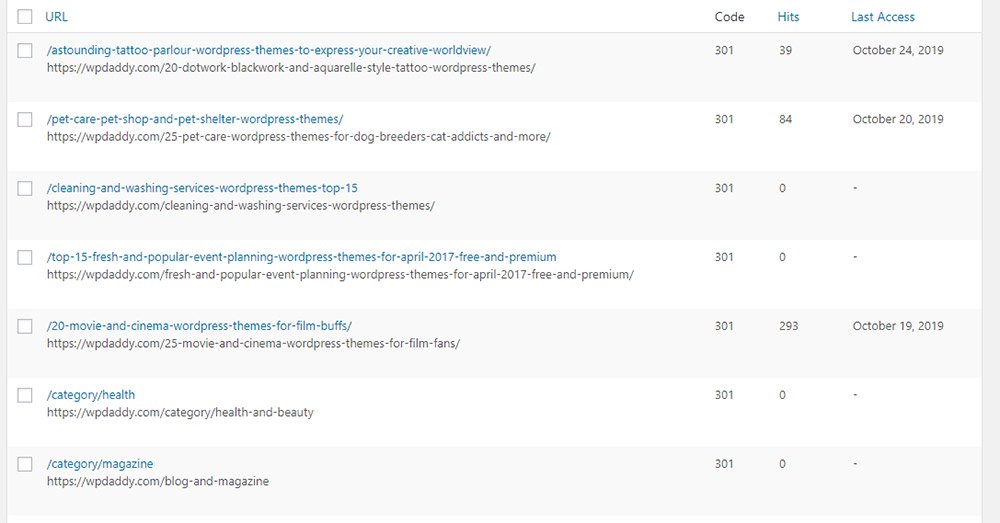A detailed view of a code analysis tool interface displays a structured table on the right side of the screen, accompanied by a graphical representation. The table categorizes data with several columns: 'URL,' 'Code,' 'Hits,' and 'Last Access,' each equipped with a checkbox extending downward for selective filtering. The 'URLs' column lists various WordPress theme categories, starting with "Tattoo Parlor Themes," followed by "Pet Shop Themes," "Washing Services Themes," "Event Planning Themes," "Film Themes," and "Health Themes." The corresponding 'Code' column uniformly shows "301," indicative of permanent redirects. 'Hits' vary across the entries, with some showing zero, while others have recorded access attempts. The 'Last Access' column indicates the latest date of data interaction, with the most historical entry logged as October 24, 2019. This detailed table offers a comprehensive snapshot of different website themes' access and interaction metrics.